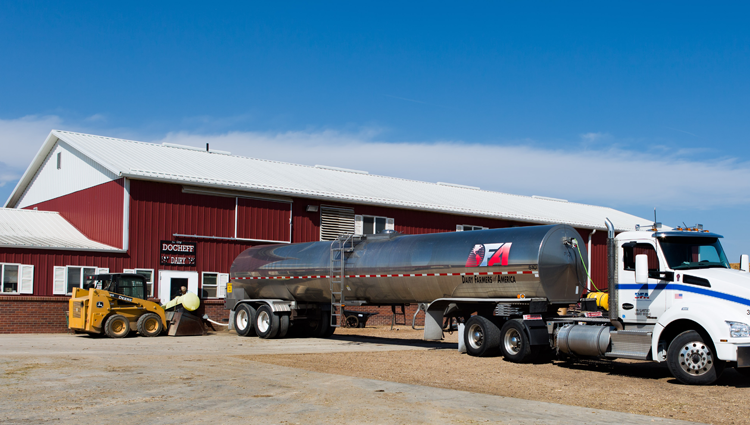The image depicts a red building with white trim and a white roof, reminiscent of a large barn, likely functioning as a small business. A sign on the building seems to read "Dog Chief Dairy," although it is not entirely clear. Attached to the building is a white gutter and several windows, one of which has white shutters. A smaller red building with white trim stands adjacent to the main structure, also featuring a white roof.

Prominently in the foreground, there is a large, silver fuel tanker truck bearing "F.A. Dairy Farmers of America" in blue and red letters, with black accents. The truck towing the tanker is white with a blue stripe. Additionally, a yellow construction vehicle, possibly a mini excavator or bobcat, is parked to the left of the truck.

The environment around the buildings consists of a stone-covered ground with spotty, possibly dead grass. Above, the sky is blue with some scattered clouds, creating a picturesque backdrop.